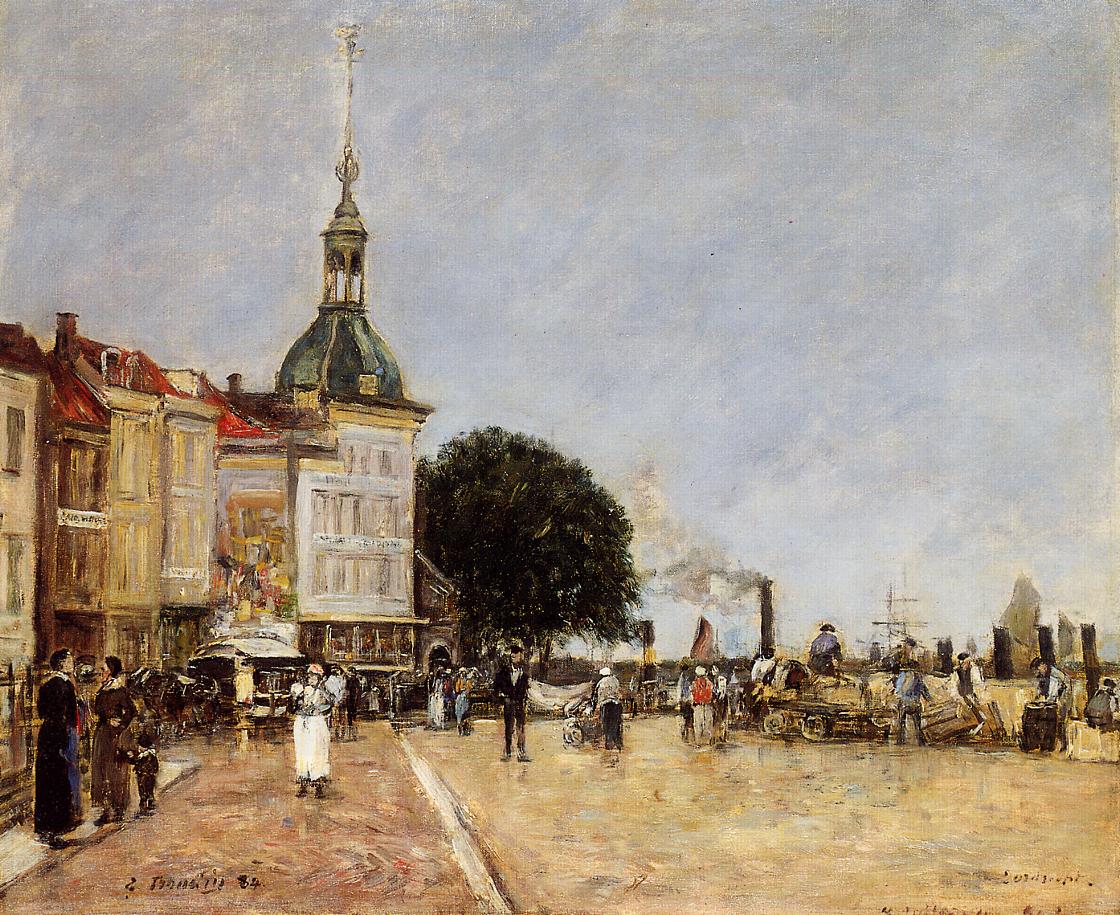This detailed impressionistic painting depicts a bustling street scene in a European city, possibly France, from the early 1800s. The foreground showcases a street painted in light beige and amber tones with hints of blue and white brushstrokes. On the left side, there is a series of three-story buildings in light yellow and brown hues. The centerpiece is a white building with a prominent green dome and a bell tower crowned by a white spire. 

In front of this building, a vibrant dark green tree stands tall. Behind it, a smokestack can be seen emitting smoke to the left. People dressed in affluent attire are scattered across the scene; a woman in a white dress walks along the orange-toned sidewalk. Nearby, a group of men is gathered around a wagon with a yellow covering and muddy wheels. 

Additionally, you can spot two individuals by the buildings on the left: one in a blue dress and another in a brown suit with a child. On the right, people are moving wooden crates near a cart. The sky is depicted with bold blue and white brushstrokes in a rough style, adding to the dynamic and impressionistic feel of the artwork. The presence of a smokestack chimney suggests a steamship or a steam engine, hinting at the proximity of a body of water just outside the frame.